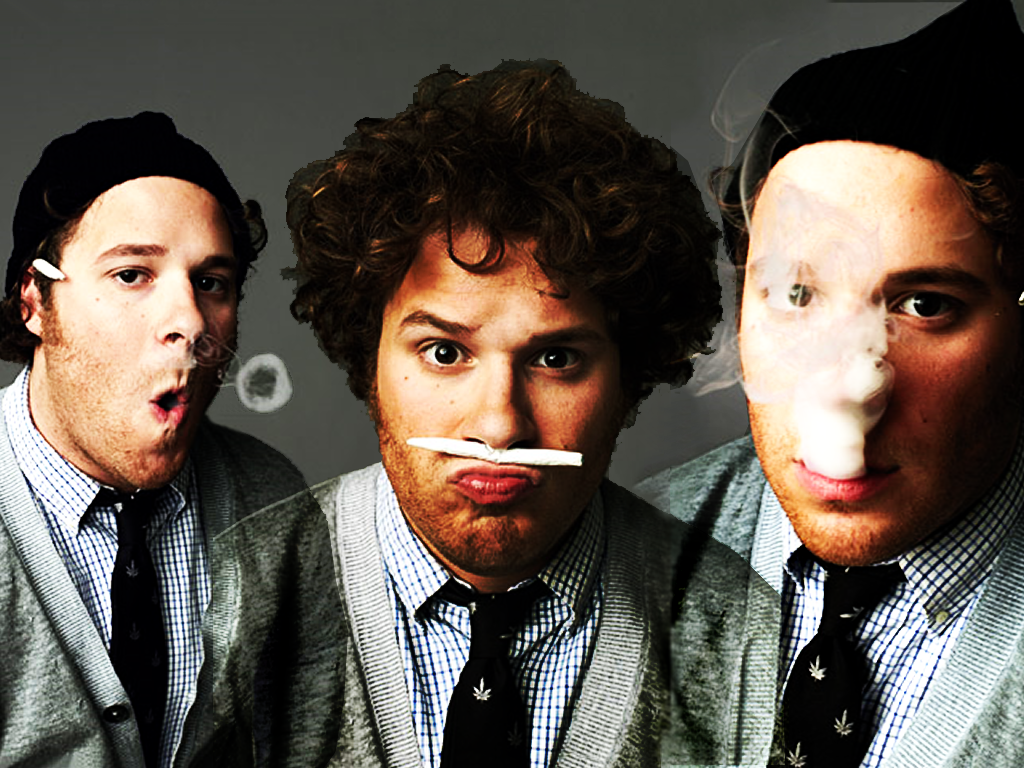The image is a triptych featuring the actor Seth Rogen, with three distinct poses against a dark gray background. All three images show Rogen dressed in a greenish-gray cardigan sweater over a white and blue striped shirt accented with a black tie adorned with marijuana leaves. His curly, thick brown hair and short stubble beard can be seen clearly in most of the shots. In the central image, Rogen balances a rolled joint between his nose and upper lip while pressing his lips together, giving a playful expression. The left image shows him wearing a beanie and exhaling a perfect smoke ring, with another joint tucked behind his ear. On the right, he also sports a beanie, but this time he is exhaling a thick cloud of smoke that obscures much of his face. The repeated elements of his attire and the smoky theme tie the images together, creating a cohesive and engaging portrayal.